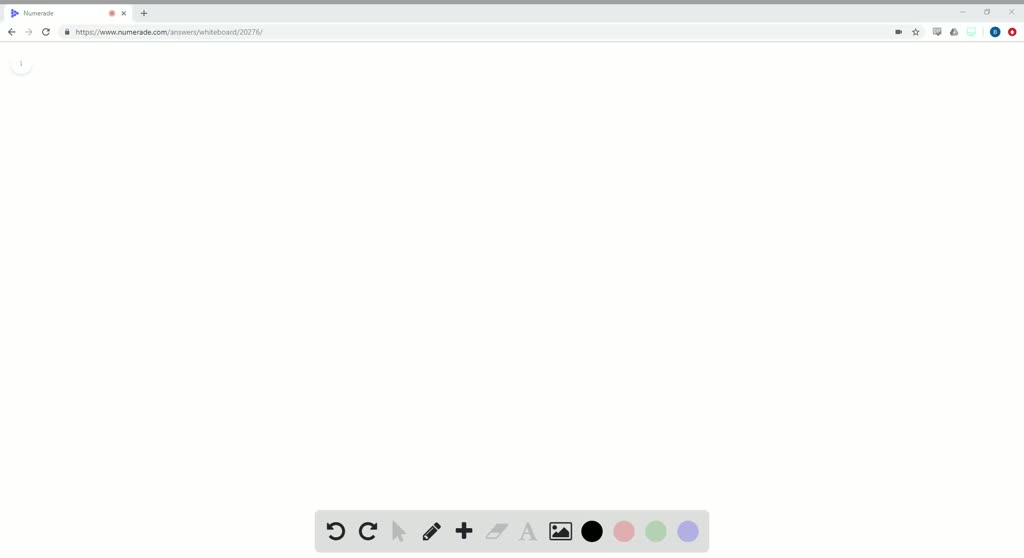In this particular screenshot, the image depicts a blank interface. At the top, there is a traditional computer menu bar with a tab currently open, featuring a blue button. Below this menu bar is a gray navigation bar that includes several icons: a back button, a forward button, a light gray arrow, an edit button, and a plus button. Additionally, there is a rectangular icon divided into a black top half and a white bottom half, followed by an unhighlighted letter 'A'. Next, there are icons of a picture, a black circle, a pink circle, a green circle, and a purple circle. The overall layout is minimalistic with a focus on the toolbar elements.